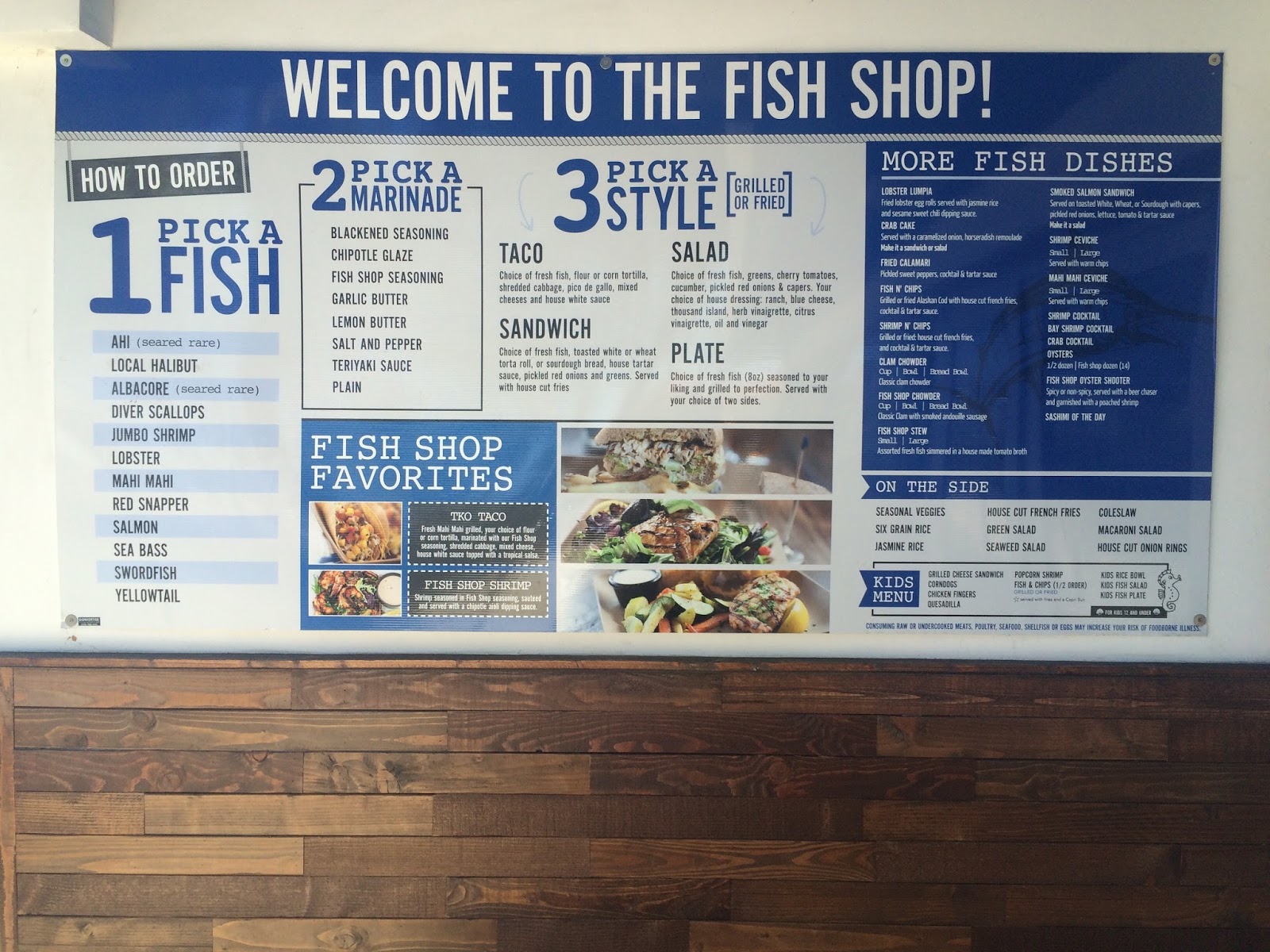The image is a full-color, horizontally rectangular photograph taken indoors at a restaurant. The wooden wall in the background, composed of brown planks, serves as a border for a prominently displayed sign. The sign itself is blue with white text and is horizontally rectangular. At the top, it warmly welcomes customers with "Welcome to the Fish Shop." Below, it provides detailed instructions on how to order: 

1. "Pick a fish" – it lists common ocean options such as salmon, lobster, and shrimp.
2. "Pick a marinade" –  options like garlic butter are provided.
3. "Pick a style" – customers can choose from taco, sandwich, salad, or plate, with the option of having the fish grilled or fried.

On the right side of the sign, there's a section for additional fish dishes and specials like calamari, as well as a kids' menu. At the bottom of the sign, labeled "Fish Shop Favorites," are enticing photos of some featured sandwiches and other fish dishes. The comprehensive and visually appealing sign guides diners through their meal choices efficiently.